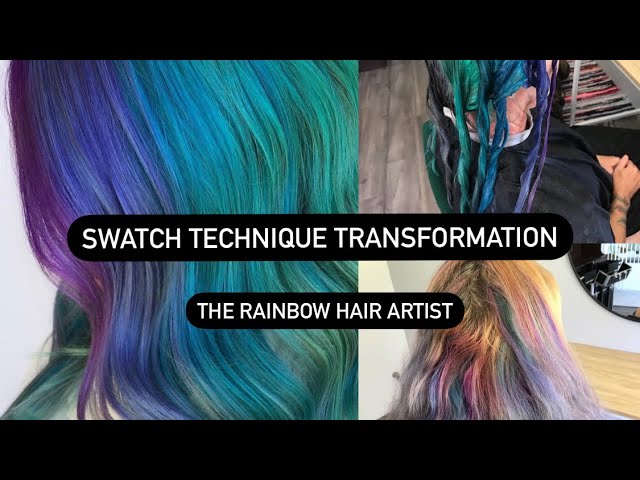This image is composed of three sections arranged in a grid. The large image on the left showcases long, multicolored hair with a stunning gradient that transitions from purple to bluish purple, then bluish, followed by green streaks, teal, and back to more green streaks. Overlaying this image are the words "Swatch Technique Transformation" in bold, white, all-caps letters. Below this text, it reads "Rainbow Hair Artist." The right side of the image features two smaller pictures stacked vertically. The top-right photo displays the hair-dyeing process: a person with hair sectioned and colored in a gradient pattern from purple at the front, transitioning to blue, then aquamarine, and finally green towards the back, while they sit with a salon cape over a wooden floor. The bottom-right photo seems to be a 'before' shot, showing hair with blonde roots and faded hints of pink, blue, and green, possibly remnants from a previous dye job. Black borders frame the entire composite image at the top and bottom.